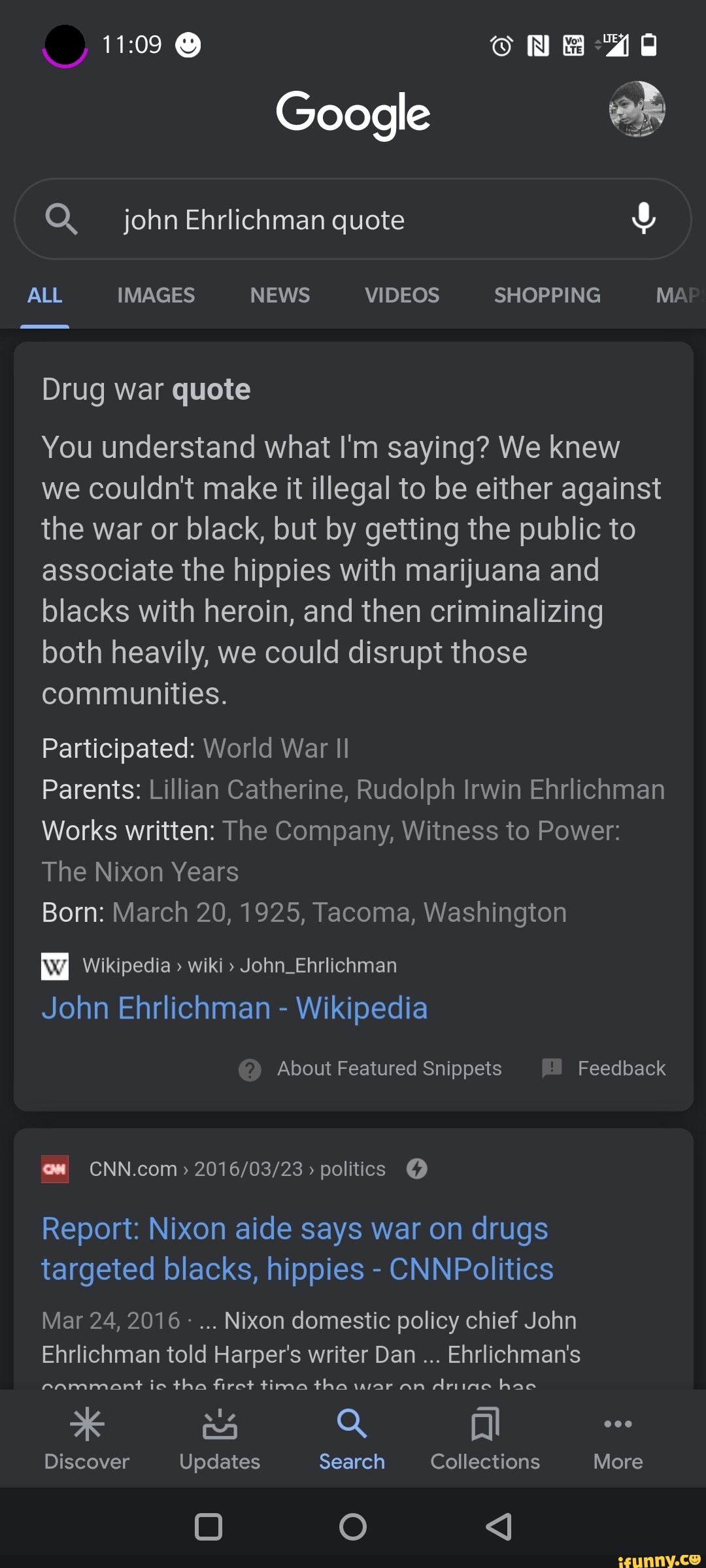The image displays a Google search page against a gray background. In the upper left corner, the time is shown as 11:09, accompanied by a smiley face icon. The upper right corner features several icons: an alarm symbol, a VOLTE and LTE data indicator, and a half-full battery icon.

Centered below is the Google logo, beneath which lies the search bar with the query "John Ilrichman quote." The navigation tabs for "All," "Images," "News," "Videos," and "Shopping" are present, with "All" being selected.

The search results include a quote attributed to John Ilrichman: "We knew we couldn't make it illegal to be either against the war or black. But by getting the public to associate the hippies with marijuana and blacks with heroin, and then criminalizing both heavily, we could disrupt those communities."

Additional information provided includes:
- Participation in World War II
- Parents: Lillian Catherine and Rudolf Irwin Ilrichman
- Written works: "The Company," "Witness Devour," and "The Nixon Years"
- Birthdate: March 20th, 1925, Tacoma, Washington

The prominent search result is a Wikipedia entry titled "John Ilrichman," highlighting a CNN Politics article "Nixon Aide Says War on Drugs Targeted Blacks and Hippies."